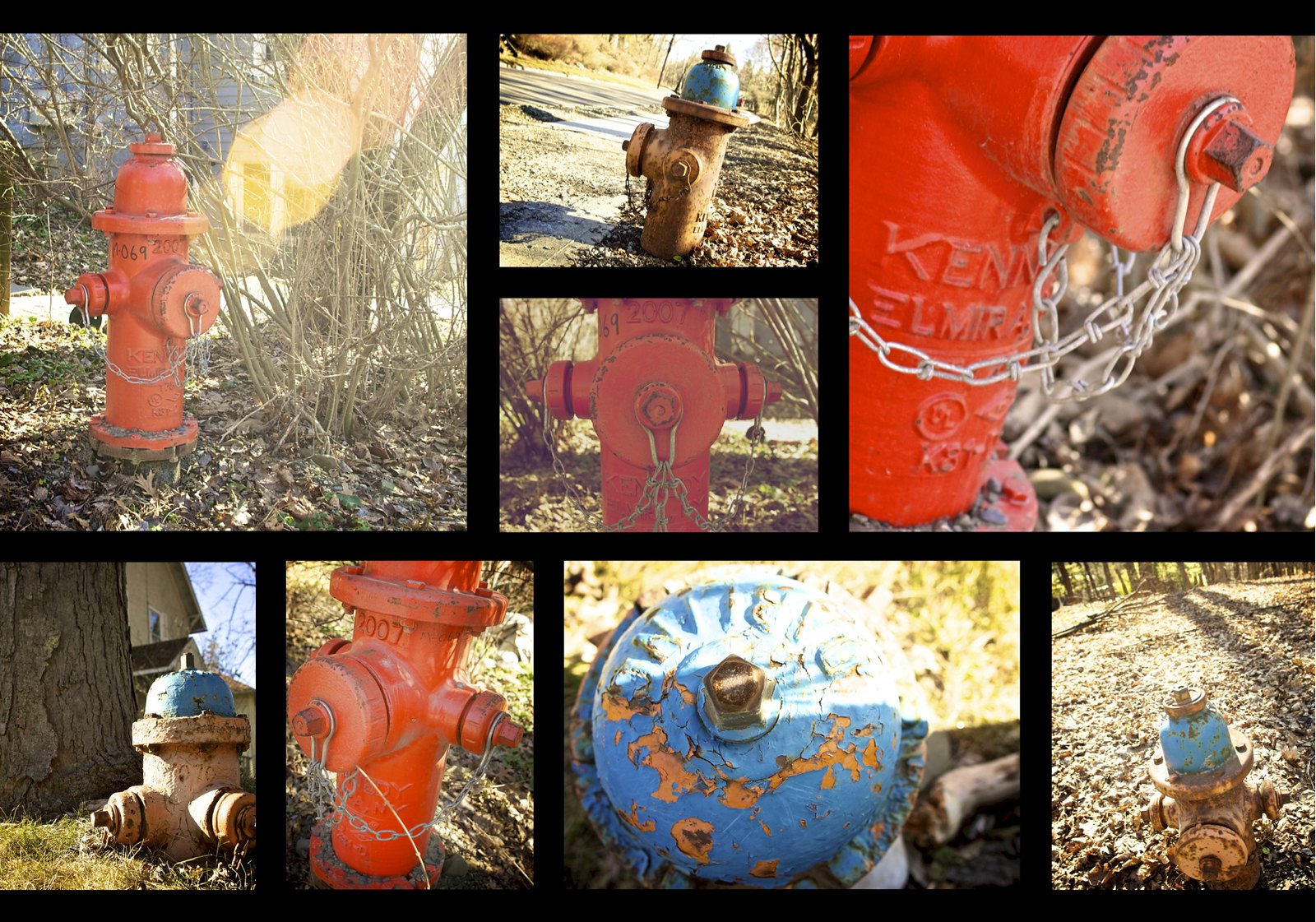This composite image showcases several photographs of fire hydrants, predominantly red, displayed in a detailed arrangement. In the upper left corner, there is a bright red fire hydrant amidst dead leaves and sticks, next to a tree with no leaves, suggesting a wintry setting. Behind it, a gray house can be seen. Moving to the right, a vertically aligned rust-orange hydrant is situated above a close-up of a red hydrant that features the text "Ken El Mira" and is adorned with silver chains. Continuing further right, there is another close-up shot illustrating the intricate details of the red hydrant with its silver chains prominently visible.

In the lower right corner, the top portion of a fire hydrant with a blue cap and rusted brown base is depicted. Adjacent to it is another image of a hydrant with a blue top and hints of rusted orange in the middle. Completing the arrangement are more hydrants along the bottom of the image: an orange rusty one, another close-up of a red hydrant, and a significantly rusted, low-lying brown hydrant with a blue top situated to the far left.